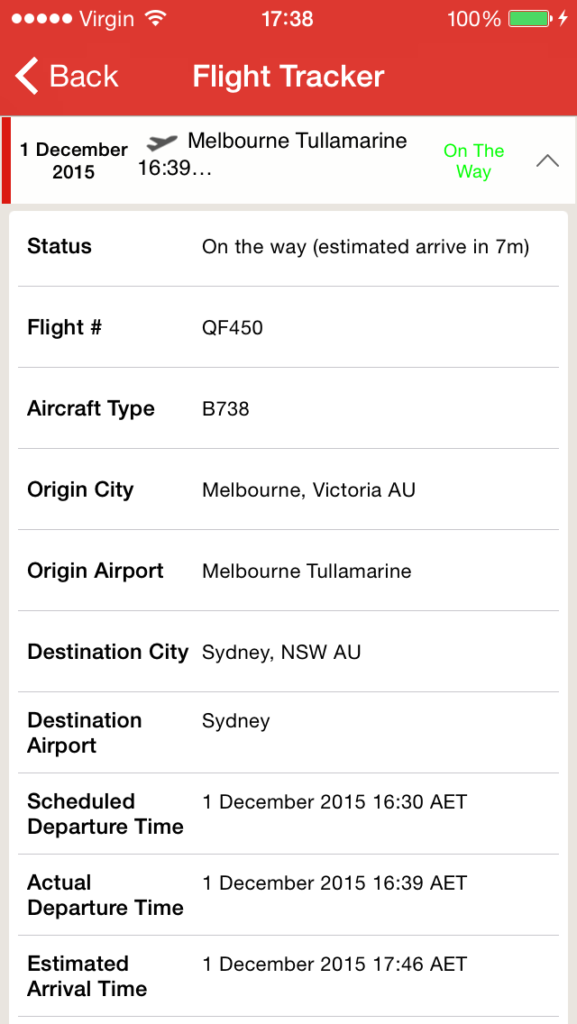A detailed caption:

A web page displayed on a smartphone shows the flight tracking details for a Virgin Airlines flight on December 1st, 2015. The flight, originating from Melbourne Tullamarine Airport (MEL) in Victoria, Australia, is en route to Sydney Kingsford Smith Airport (SYD). The flight's status is "On the way," with an estimated arrival time of 17:46. The scheduled departure time was 16:30 AEDT (Australian Eastern Daylight Time), but the actual departure was at 16:39, making the flight nine minutes behind schedule. The estimated flight duration is approximately 1 hour and 7 minutes. The tracker provides comprehensive information, including the flight number and aircraft type, to keep travelers and those awaiting passengers informed about the flight's progress.